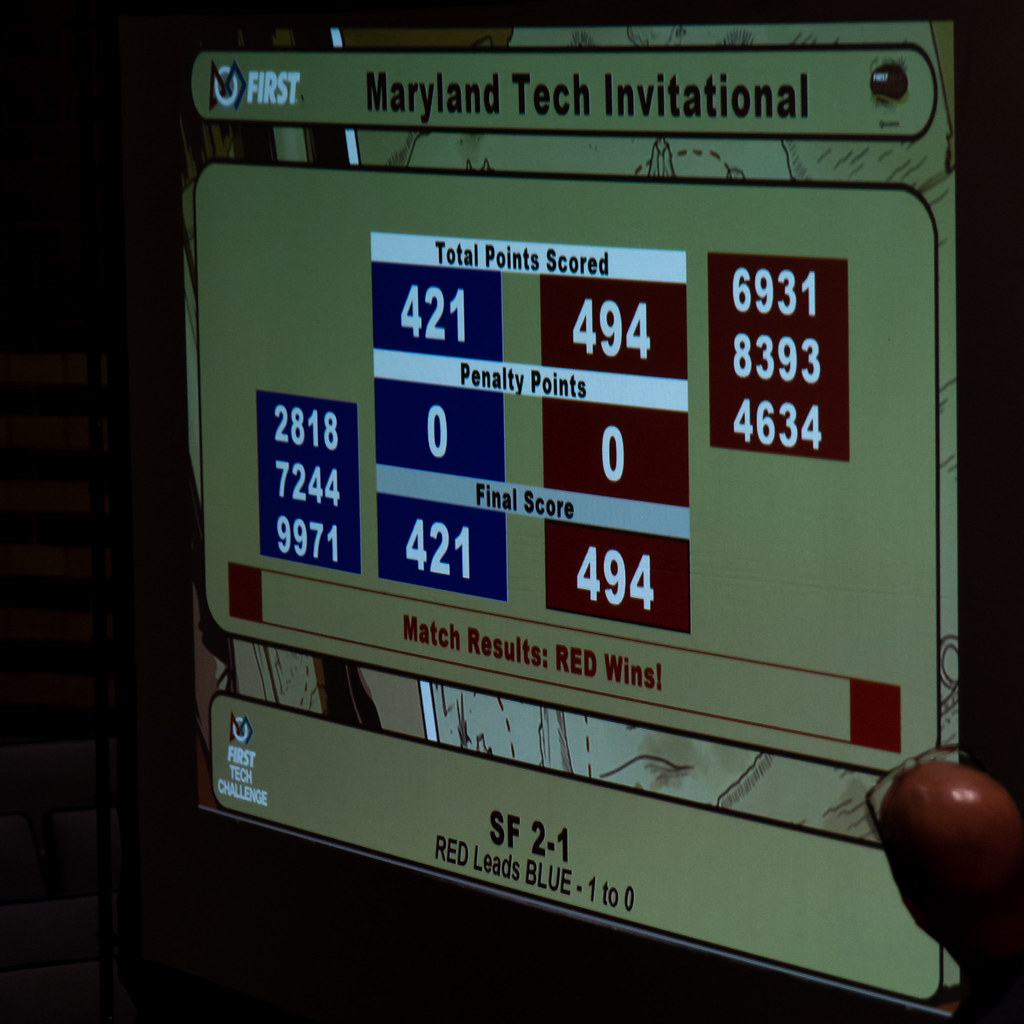The image features a projection screen displaying detailed results from the Maryland Tech Invitational. At the top, within a green circular rectangle, it reads "First Maryland Tech Invitational." Below, the screen is divided into two columns indicating team scores. The left, representing the blue team, displays the total points scored as 421, while the red team on the right scored 494, leading to the final result of red winning with 494 points over 421. There were zero penalty points for both teams. Below the point totals, blue team members' scores are listed as 2018, 72, 44, 99, and 71, versus the red team members' scores of 69, 31, 83, 93, and 46, 34. The results text box at the bottom confirms "match results: red wins" with the details "SF 2-1, red leads blue 1-0." In the bottom right corner of the image, there's a partial view of a balding person wearing glasses, reinforcing the impression of a live event possibly being projected.